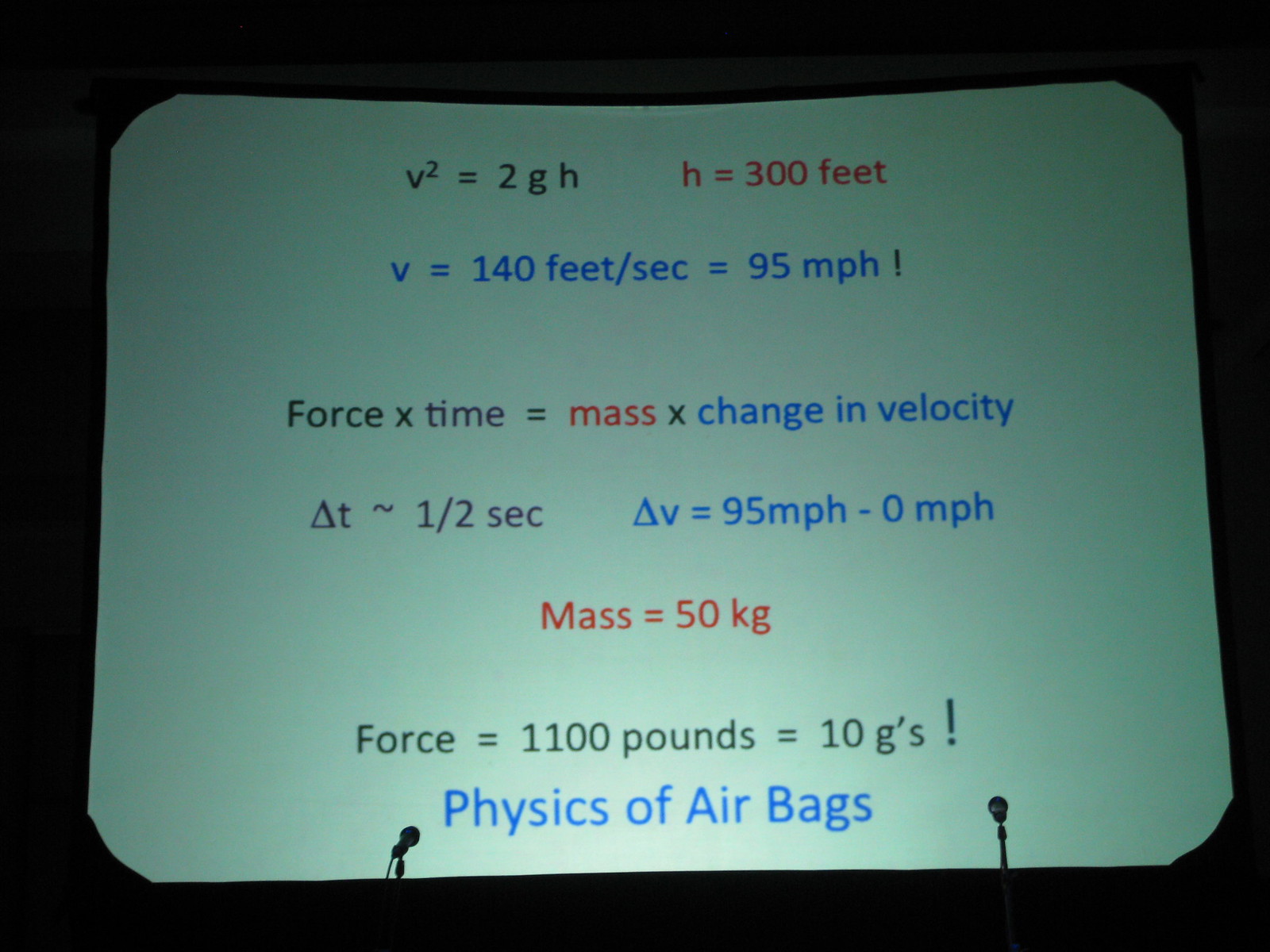In a dark room, a large projector screen displays a detailed slide filled with physics equations, with two microphone silhouettes standing in front of it. At the top of the screen, white text reads "v² = 2gh" and "h = 300 feet." Below that, in blue text, it states "v = 140 feet/second = 95 miles/hour!" The subsequent equation, "force x time = mass x change in velocity," is followed by "Δt ≈ 0.5 seconds" and "Δv = 95 miles/hour - 0 miles/hour." Further down, it notes "mass = 50 kg," and "force = 1100 pounds = 10 G's!" The bottom of the slide, also in blue, reads "Physics of Airbags." The room's darkness highlights the vivid colors of the equations and the screen, creating a stark contrast with the silhouettes of the microphones at the bottom, suggesting a presentation or lecture setting. The overall scene emphasizes the calculations involved in the physics of airbags, possibly for an educational or professional demonstration.